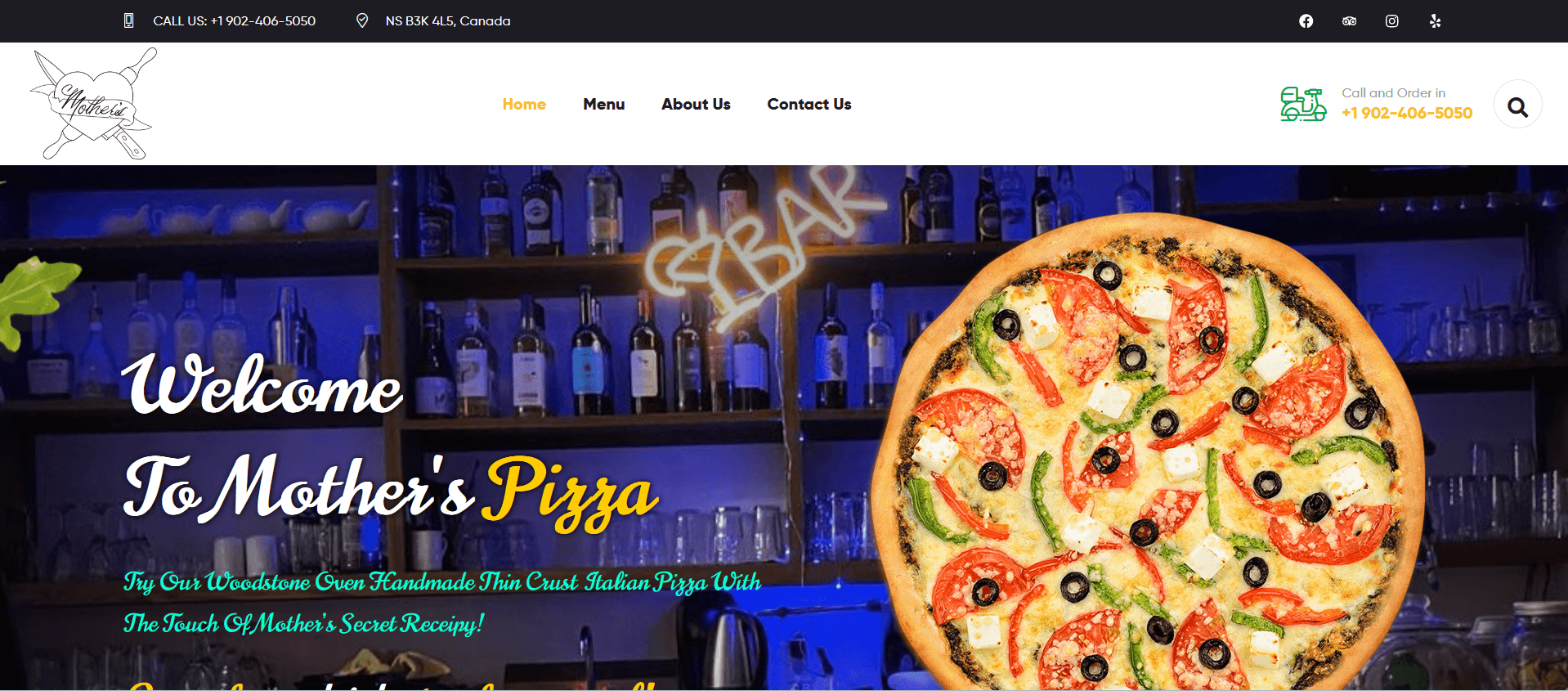The webpage for "Mother's Pizza" features a hierarchal and streamlined navigation interface. At the very top, there is a menu bar with links to the "Home," "About Us," and "Contact Us" pages, making it easy for visitors to explore the website. In the upper-right corner, users can find social media icons, including Facebook, along with a contact number with a 902 area code, offering a quick way to reach the restaurant.

The main content of the page prominently displays an inviting image of the restaurant's bar, showcasing shelves stocked with a variety of bottles. Dominating the center of the page is a warm welcome message for Mother's Pizza. The text encourages visitors to try their Woodstone Oven Handmade Thin Crust Italian Pizza, highlighted with "The Touch of Mother's Secret Recipe," although there is a small typo in the word "recipe" (misspelled as "receipy").

Accompanying the welcome message is a mouthwatering image of the featured pizza, adorned with fresh tomato slices, red and green peppers, olives, and wedges that appear to be Parmesan cheese. The overall presentation emphasizes a cozy, inviting atmosphere, suggesting that Mother's Pizza is a delightful place to enjoy a delicious meal and a relaxed dining experience.